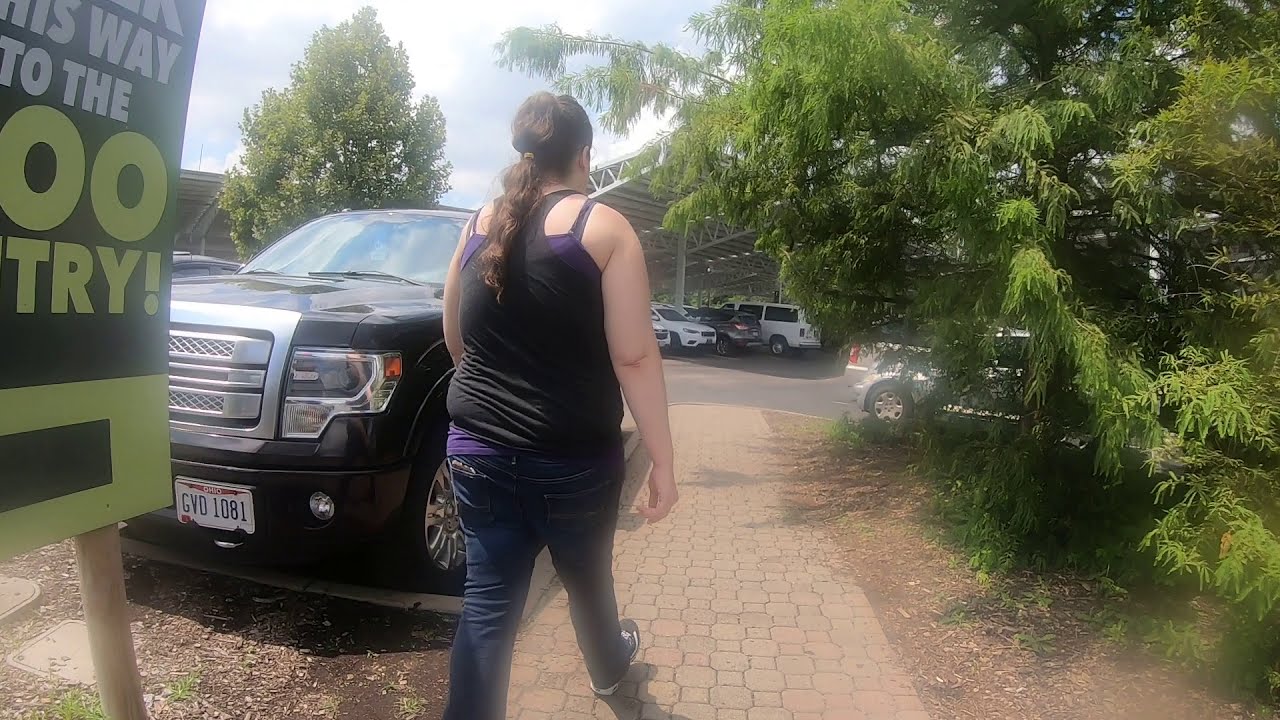This wide, horizontally-aligned rectangular image captures the backside of a woman walking away from the camera on a small stone path made of light brown cobblestones. She wears a black tank top over a purple one, blue jeans, and sneakers. The woman has white skin, a brown ponytail, and appears slightly overweight. To her left is a black Ford pickup truck with a license plate reading GVD1081, likely from Ohio. There is a partially visible green and white sign nearby indicating directions with the words, "way to the," and "00," with an arrow pointing to the left. 

The path is flanked by mulch and dirt, leading to a parking area. On the left, wood poles are partially visible, while on the right, several large green trees with leaves are evident. The sky above is mostly sunny with some gray clouds allowing beams of sunlight to poke through. Beyond the trees and towards the background, a cluster of cars is parked, including across the street and partially obscured on the right side. The setting might hint at a zoo or a similar recreational area, adding context to the composition.